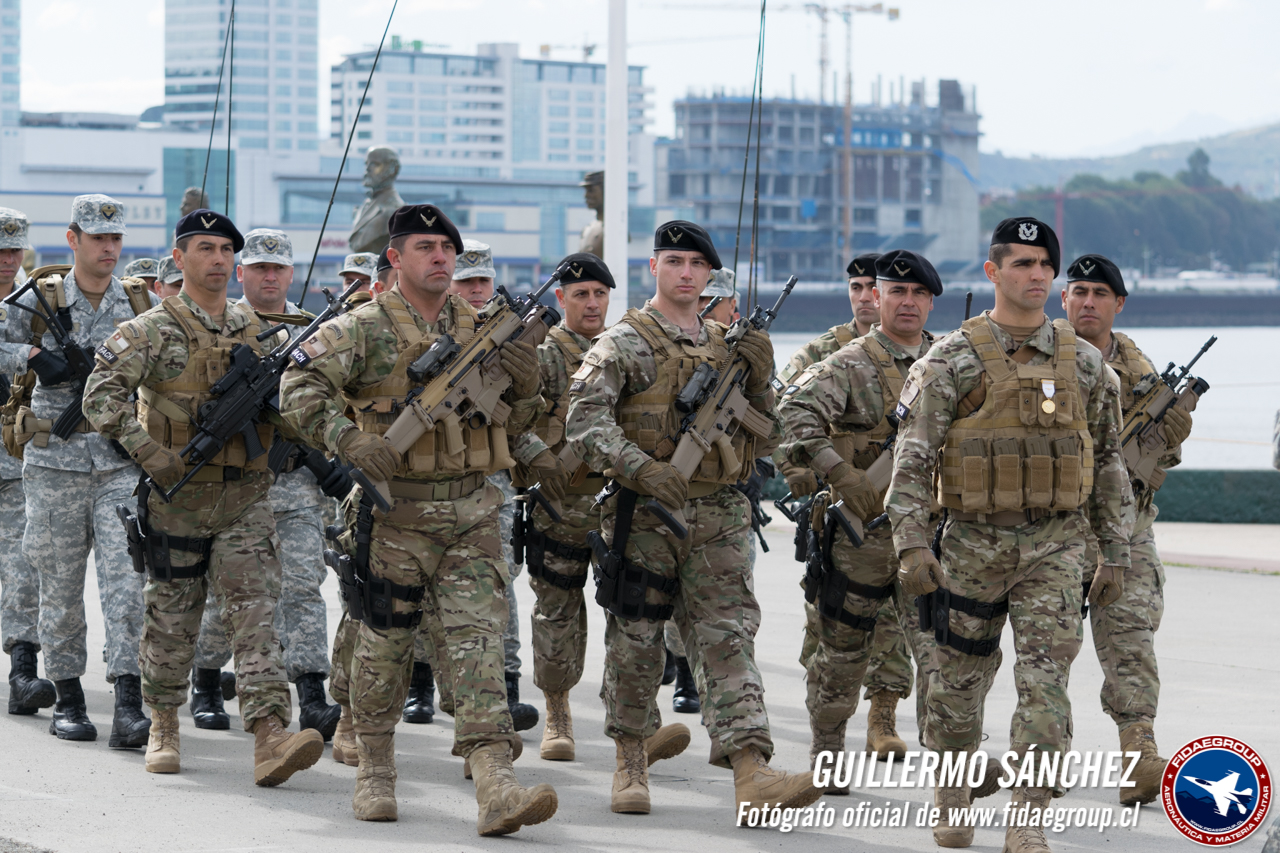The photograph depicts a group of military men, predominantly in their 30s and 40s, marching in an orderly formation along what appears to be a port area with a small or large body of water in the background. These men are clad in varied camouflaged uniforms; those in the front don darker attire compared to the lighter uniforms seen towards the back. Each man wears a black beret, a bulletproof vest equipped with pockets likely meant for ammunition or other supplies, and combat boots. A striking detail is the black band around their thighs. They are armed with large automatic rifles and appear to be walking in four organized lines. In the distance, tall skyscraper buildings, possibly both residential and commercial, form the skyline. In the bottom right corner of the image, there is text in Spanish that includes the name "Guillermo Sanchez," a symbol resembling an airplane, and the URL "www.fideigroup.cl," hinting that the men may not be part of the American military. The caption at the bottom reads: "Guillermo Sanchez, fotografo oficial."